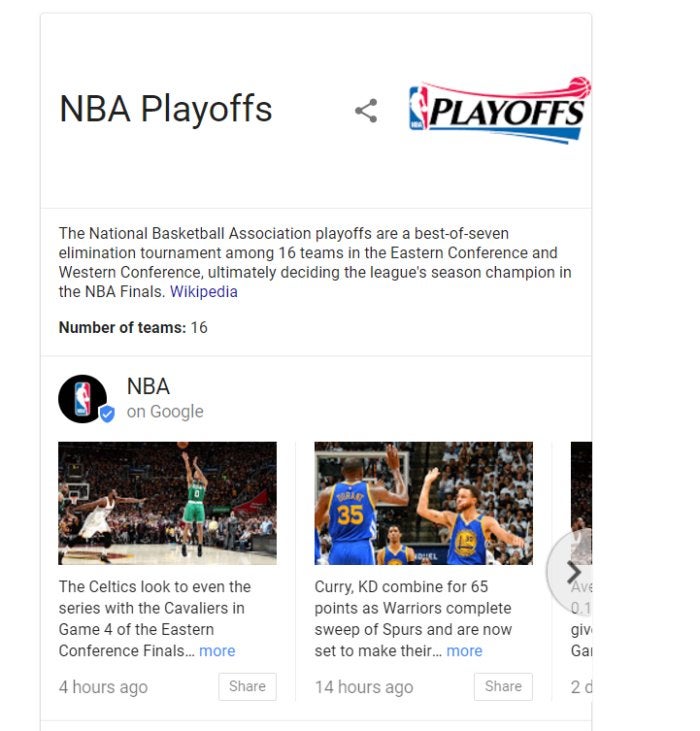The image appears to be a screenshot from a digital device, possibly a web page or a mobile phone. At the top left of the screen, the words "NBA Playoffs" are displayed prominently. In the center, there's a small half-triangle link icon, followed by the official NBA Playoffs logo on the right side.

Beneath these elements, a detailed text box explains, "The National Basketball Association Playoffs are a best-of-seven elimination tournament among 16 teams in the Eastern Conference and Western Conference, ultimately deciding the league's season champion in the NBA Finals," attributed to Wikipedia. 

Below this text, there's information specifying the "Number of teams: 16." Under a slight dividing line, the NBA logo is present alongside a blue checkmark, labeled "NBA on Google." 

Two photographs appear beneath this section. The first image on the left depicts a Boston Celtics player shooting a basketball during a game. The second image captures a Golden State Warriors player in action. A partially visible third image is cut off by the screen, and a half-bubble arrow icon indicates that more content can be viewed by scrolling or clicking further.